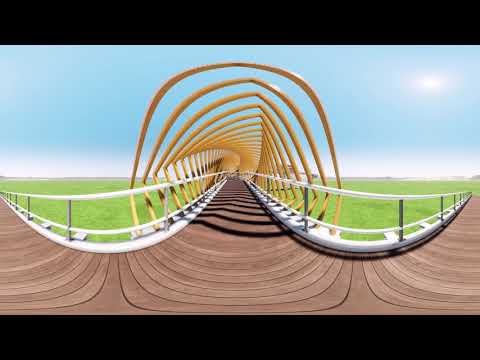This image depicts an animated or video game scene featuring an extensive deck-like walkway extending into the distance, flanked by a white railing. An almost yellow, metal pipe winds along and around the walkway, contributing to an intricate, geometric design. Captured in a 360-degree camera setting, the image appears digitally constructed rather than photorealistic, evidenced by the warping effects and animated aesthetic.

The walkway, adorned with wooden planks, stretches out under a clear blue sky, devoid of clouds. At the top and bottom of the image, there's a black rectangular framing, enhancing the surreal nature of the scene. Far in the distance, grassy fields are visible, and fleeting glimpses of hills or mountains break the horizon. Additionally, a decorative overhead structure – possibly part of the railing system – frames the path beneath it, adding to the image's animated charm. The daytime setting and the unobstructed horizon further highlight the surreal and expansive landscape.